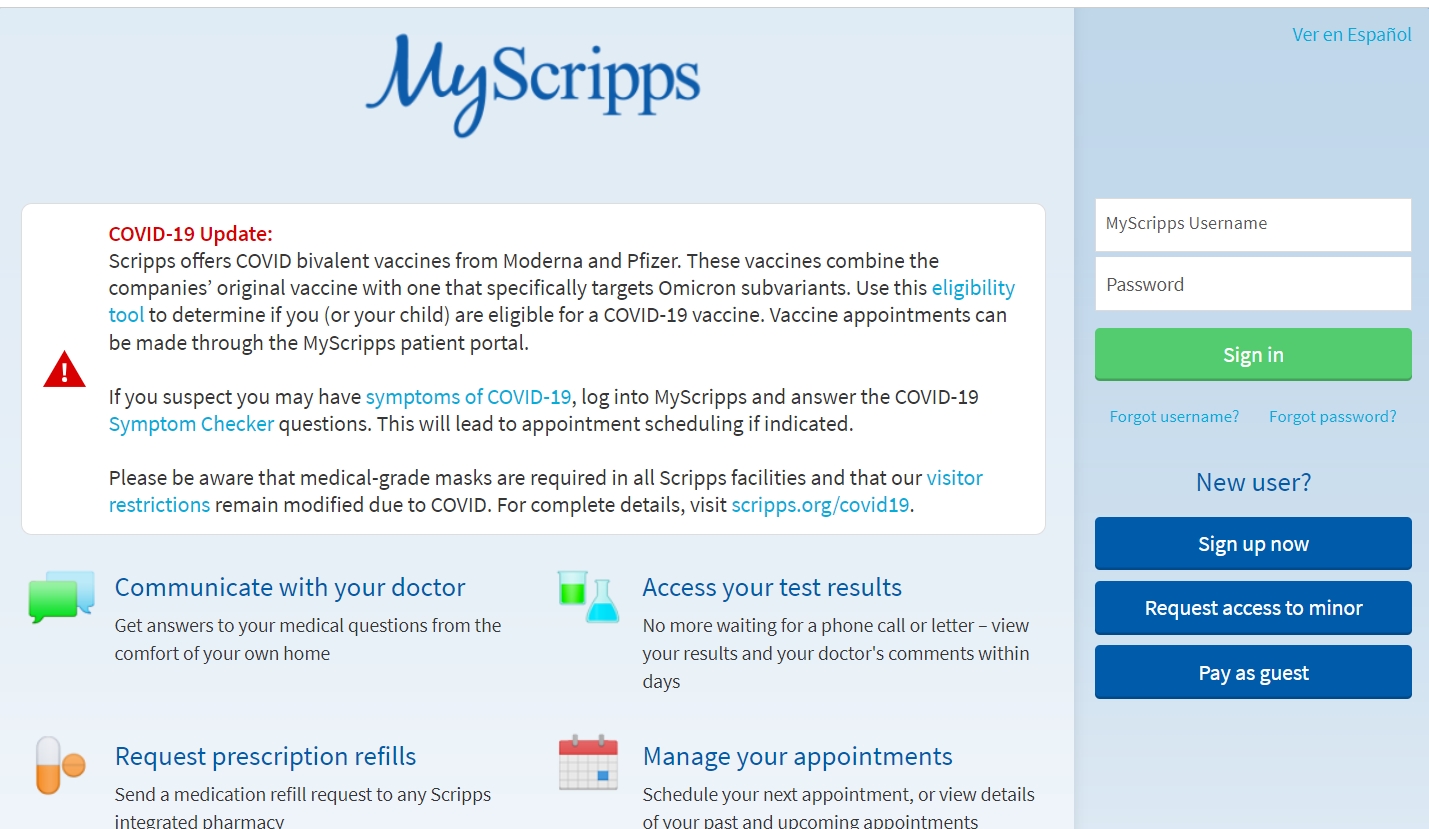**Caption: MyScripts Login Page with COVID-19 Vaccine Information**

The screenshot displays the MyScripts login page, which features a sleek and organized design in varying shades of blue with white accents. The MyScripts logo is prominently centered at the top, featuring "My" in a slightly italicized font and "Scripts" in a print font, colored in darkish blue against a very light blue background.

On the right side, a vertical light blue rectangle contains an option to switch languages, labeled "Ver en Español" in bright blue.

Below the logo, the login section consists of two text boxes labeled "MyScripts Username" and "Password," both placed on a white background. A lime green "Sign In" button with white text is positioned beneath the text boxes. Further down, two blue links say "Forgot Username?" and "Forgot Password?" A darker blue link labeled "New user?" is accompanied by three dark blue buttons: "Sign Up Now," "Request Access to Minor," and "Pay as Guest."

To the left, a white rectangular information box pops against the pale blue background. A red triangle with a white exclamation point at the top signals a critical update on COVID-19. The update text reads:
- "COVID-19 Update: Scripps offers COVID bivalent vaccines from Moderna and Pfizer. These vaccines combine the company's original vaccine with one that specifically targets omicron subvariants. Use this eligibility tool to determine if you or your children are eligible for a COVID-19 vaccine. Vaccine appointments can be made through the MyScripts patient portal.
- If you suspect you may have symptoms of COVID-19, log into MyScripts and use the COVID-19 Symptom Tracker. This will lead to appointment scheduling if indicated. 
- Please be aware that medical-grade masks are required in all Scripps facilities, and visitor restrictions remain modified due to COVID. For complete details, visit scripps.org/covid19."

The lower section features four informational icons:
1. Two chat bubbles (green and lime green, and bright blue) with the text "Communicate with your doctor." Below it, in black, it reads, "Get answers to your medical questions in the comfort of your own home."
2. Two beakers, one lime green and one bright blue, with the text "Access your test results." Underneath, it states, "No more waiting for a phone call or letter—view your results and your doctor's comments within days."
3. An icon with a white and orange pill next to an orange round pill, accompanied by the text "Request prescription refills." Below, it says, "Send a medication refill request to any Scripps integrated pharmacy."
4. A red and white calendar icon, labeled with "Manage appointments." It explains, "Schedule your next appointment or view details of your past and upcoming appointments."

This comprehensive layout not only facilitates user interaction but also provides essential updates and functionalities to ensure patients can efficiently manage their healthcare needs and stay informed about COVID-19 protocols.